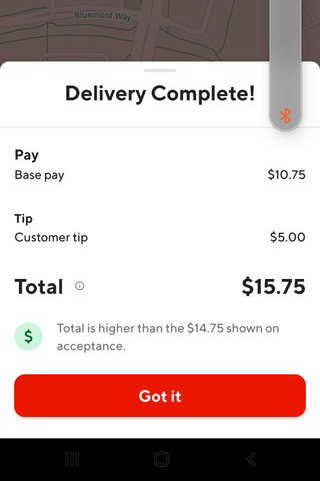The image displays a section of a map with the top portion grayed out, revealing the text "Bluemont Way" within the gray area. A vertical, rounded bar featuring the Bluetooth logo in orange appears prominently. Centered on the image is a white box with a gray border containing bold black text declaring, "Delivery Complete."

Below this text is a horizontal bar. To the left of this bar, the word "Pay" is printed in bold black letters, followed by the text "Base Pay" immediately underneath. To the right of this, the amount "$10.75" is displayed. Beneath this section, in bold type, the word "Tip" is written followed by "Customer Tip: $5." 

Further down in the largest typography, the word "Total" is placed next to a small gray circle with an 'i' symbol inside. To the right, the total amount "$15.75" is shown. Directly below this, there is a green circle featuring a darker green dollar sign, accompanied by the text, "Total is higher than the $14.75 shown acceptance."

At the bottom of the image, a horizontal red rectangle with rounded corners is inscribed with the words, "Got It." The very bottom features a black bar with no text.